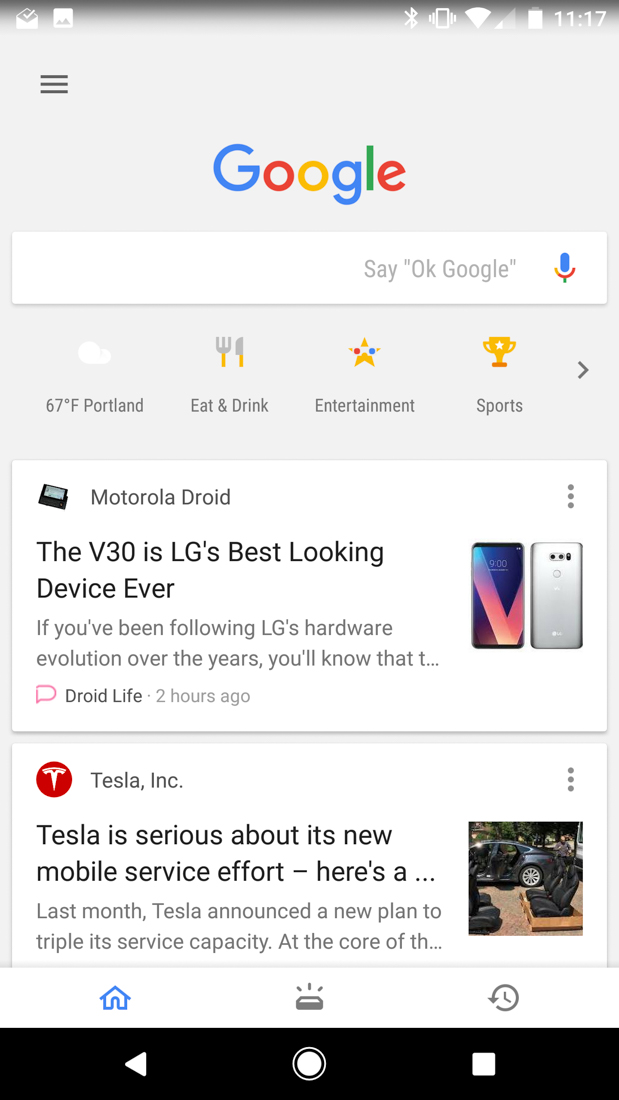A detailed caption of the smartphone screenshot:

---

The screenshot captures the results from a Google search on a Motorola Droid smartphone. The device’s screen displays various icons: a photo icon, Bluetooth icon, vibration mode, Wi-Fi signal strength (less than half full), and the battery icon indicating it is 11:17 AM. The Google logo is prominently featured at the center top of the display, with a hamburger menu icon situated to the upper left.

Beneath the Google logo, the search field is showcased with an instruction to "Say 'Ok, Google'", accompanied by a microphone icon. Below this search bar, the weather widget displays a current temperature of 67 degrees Fahrenheit in Portland. 

Following the weather information, there are various categorized sections such as "Eating & Drink", represented by a knife and fork icon; "Entertainment," symbolized by a gold star with blue and red dots; and "Sports," marked with a trophy icon. To the right of these sections, there's an arrow indicating more options.

The search results begin with a description of the Motorola Droid V30, highlighted as LG's best-looking device ever, including front and back images of the phone sourced from Droid Life, posted two hours ago. Following this, another search result features Tesla Inc., discussing the company's new mobile service effort, with reference to an announcement about tripling its service capacity. This result includes an image of a Tesla car and several seats placed outside on the ground next to a pallet.

Below the search results and on the device's home screen are buttons for Inbox and a rewind icon, along with a black bar at the bottom of the screen featuring a navigation menu.

---

This enhanced description provides a clear and thorough account of the elements visible on the smartphone's screen.